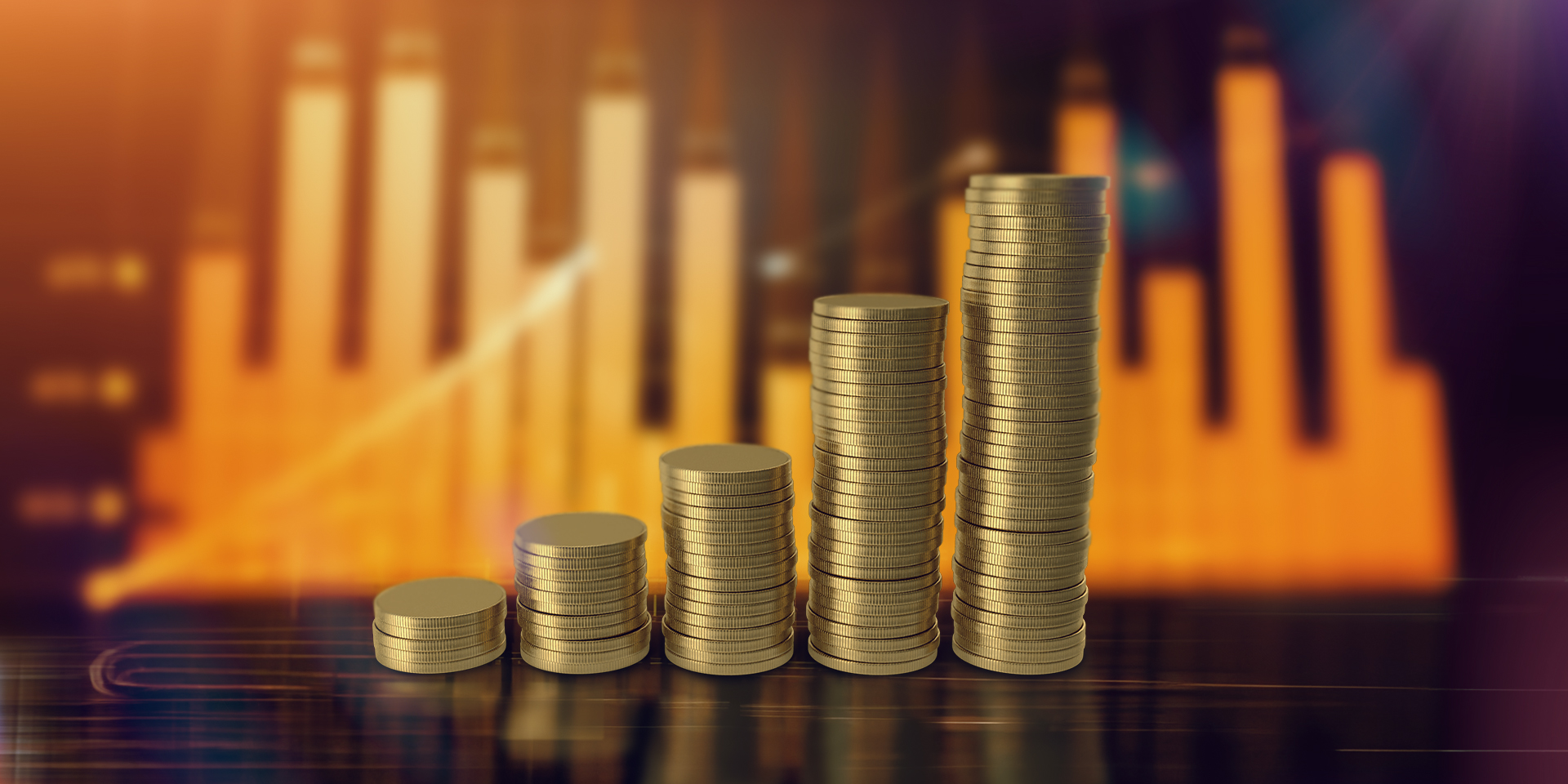The photograph depicts five rows of gold-colored coins, each stack taller than the previous, lined up like ascending steps from left to right on a sleek, black shiny wooden table. In the blurred background, there is a chart with orange bars of varying heights, similar to a bar graph or financial chart, that fluctuate up and down in an irregular pattern. Despite the lack of clarity, the chart's colors are mostly golden yellow, occasionally appearing to resemble buildings, and feature purple and blue hues. The coins are centrally positioned in the image, creating a strong contrast against the reflective surface below.